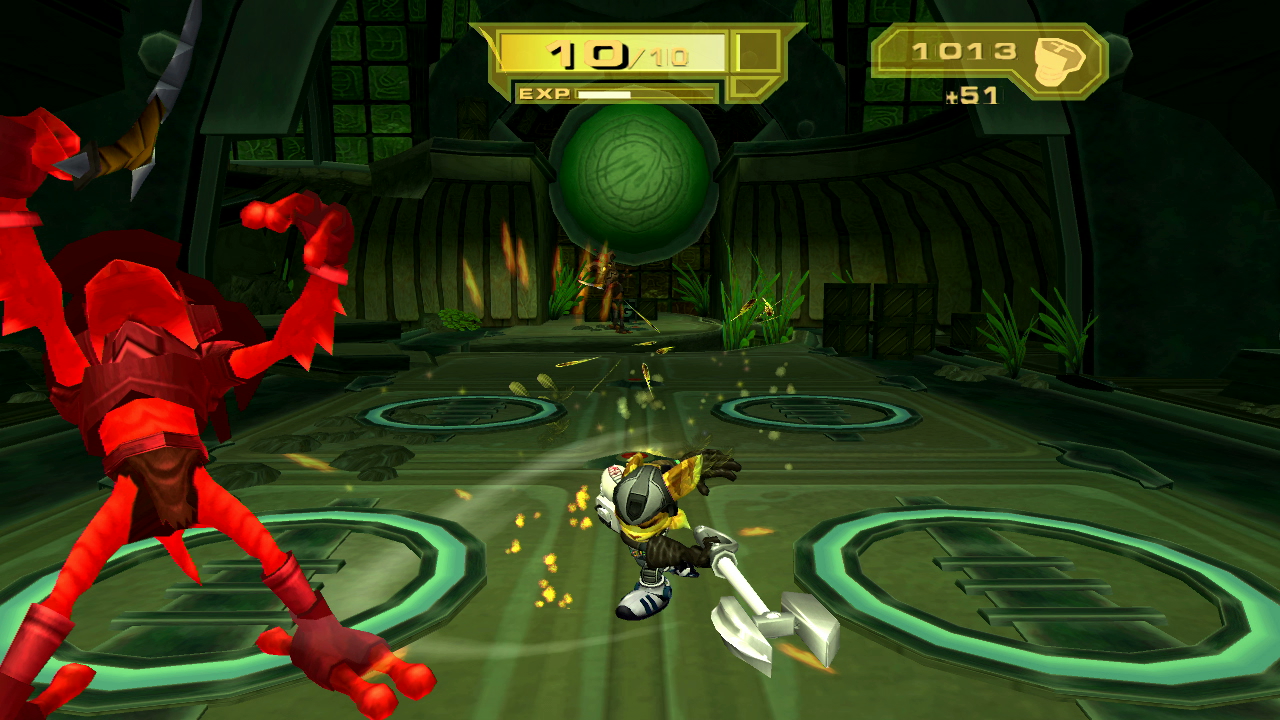This screenshot from a video game showcases a vibrant green playing field segmented into four rectangular parts with numerous circular elements scattered throughout. At the center, there's a distinctive green circle at the far end. Detailed graphics depict green grass interspersed with fiery accents. 

Two anthropomorphic characters dominate the scene: on the left, a humanoid cat dressed in casual clothes and sneakers, wielding a long, cylinder-like arm ending in metal claws. On the right, a large red creature with clawed feet and crab-like pincers stands prominently, facing away from the camera with its arms raised. 

Additional elements include a helmeted yellow creature carrying a labrys running down the center of the field, and a flexing red figure at the bottom left suggesting a complex interactivity. At the top right, a square displays the number "2013" and a bolt icon accompanied by "+51". An experience bar, a life bar indicating "10 out of 10", and a score displaying "1013" are also featured, enhancing the immersive gameplay interface.